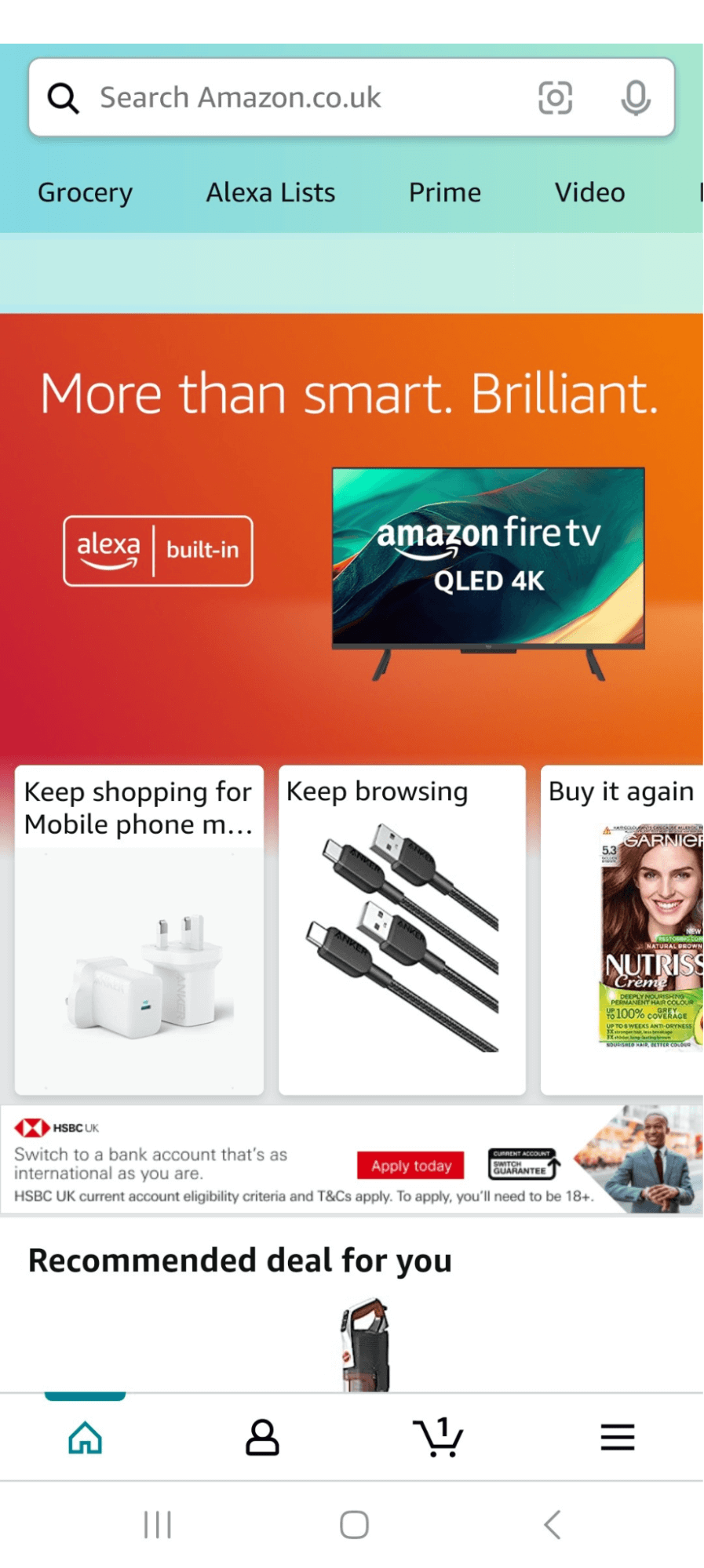This screenshot captures an Amazon.co.uk webpage, providing a comprehensive view of various site elements and promotional materials. At the top, the page features a search bar labeled "Search Amazon.co.uk," complemented by a magnifying glass icon to the left and camera and microphone options to the right. Just below this search bar, several categories are displayed horizontally, specifically: Grocery, Alexa List, Prime, and Video, all set against a backdrop in a teal or Tiffany Blue hue.

Dominating the center of the page is a prominent advertisement boasting the slogan "More Than Smart. Brilliant." This ad highlights an Amazon Fire TV with QLED 4K, including a note that the device has Alexa built-in. Beneath this main banner is a segment encouraging continued shopping for mobile phone accessories. This section showcases an assortment of outlet chargers and cable management products.

Further down, the page suggests products to "Buy it again," featuring a specific hair coloring product. Lastly, at the bottom of the screenshot, there is an advertisement for HSBC UK, promoting their current account services with the slogan, "Switch to a bank that is as international as you are." The fine print clarifies that eligibility criteria and terms and conditions apply, noting that applicants must be 18 years or older.